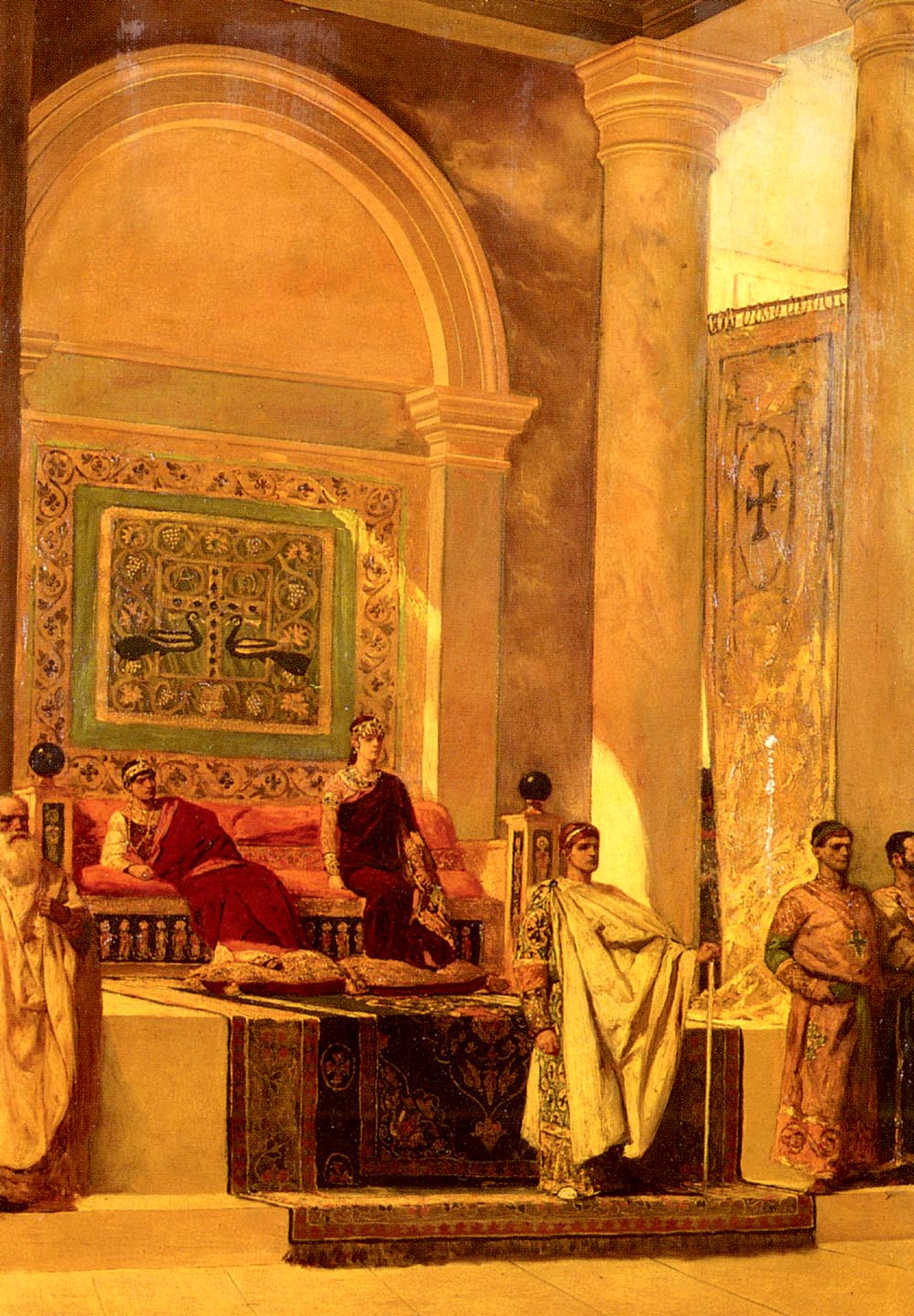This painting depicts an ancient royal scene, likely set in a Roman or possibly Egyptian interior. Dominating the composition is an elevated area adorned with oriental rugs and tapestries, upon which a king and queen are seated on a regal, long futon-like couch. The king, with legs crossed and a relaxed demeanor, contrasts sharply with the queen, who sits upright, poised as if awaiting someone. Their attire and the ornate design of their robes highlight their royal status.

Around the central figures stand several individuals in toga or robe-like garments. To the left, an elderly man with a white beard appears more distinguished. A prominent robed guard, holding a staff, stands near the center, flanked by two other men whose simpler robes indicate lower status. All the figures seem focused on something beyond the right edge of the painting.

The background features a vivid tapestry with green patterns that resemble birds, and to the right, a large golden banner displaying a cross. The predominant colors in the painting are yellow, orange, and green, which add a warm, vibrant feel to the scene. Overall, this artwork richly captures a moment of royal anticipation or reception within a grand historical setting.